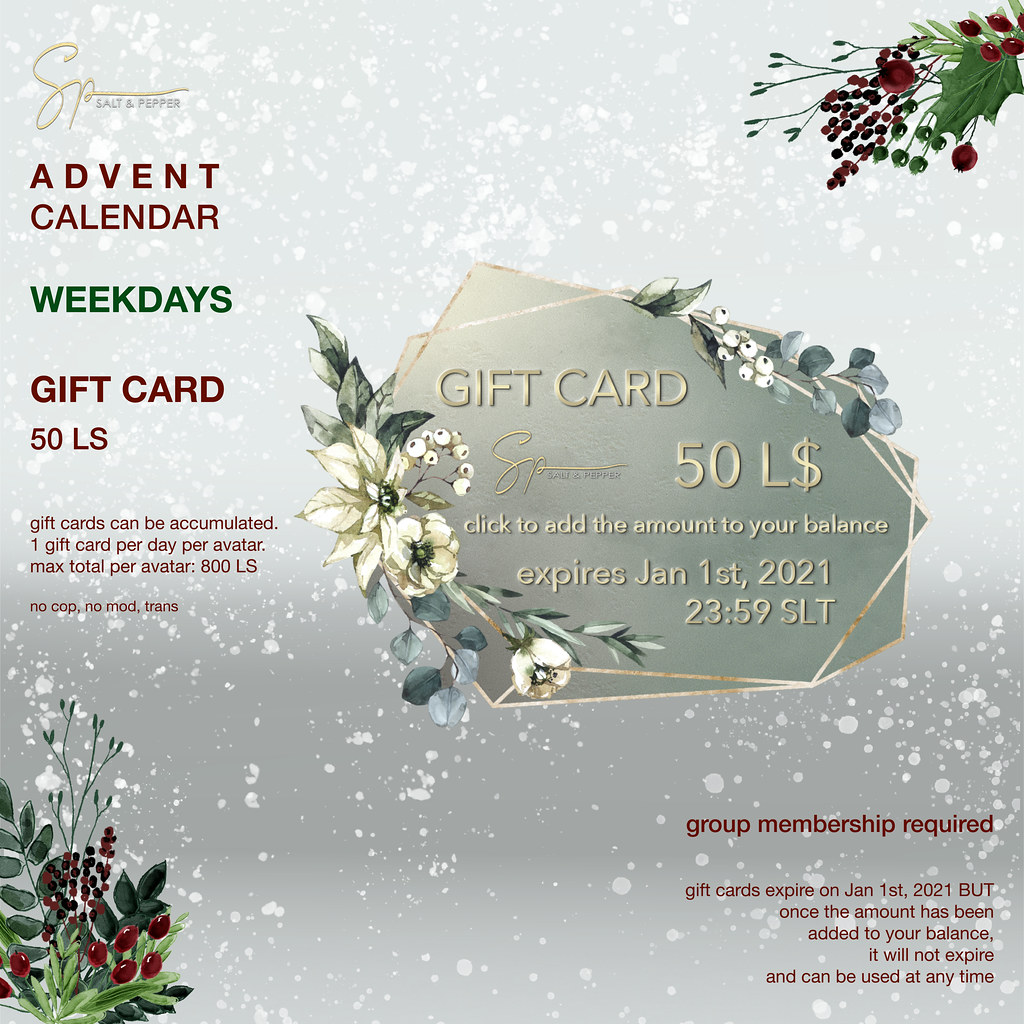The image is a digitally synthesized advertisement for Salt & Pepper's Gift Card Advent Calendar. The background fades from light to dark gray, dotted with white speckles mimicking snow. 

In the top left corner, the brand's logo, "SP" in gold cursive, leads into "Salt and Pepper" in small gray font. Beneath it, "Advent Calendar" is displayed in bold maroon block text followed by "Weekdays" in green. Continuing below in maroon, "Gift Cards 50 LS" is noted, with a detailed explanation: "Gift cards can be accumulated, one per day per avatar, with a maximum total of 800 LS per avatar. No cop, no mod trans."

Both the top right and bottom left corners feature clip art of holly and other Christmas plants, in dark green and red. Midway on the right, a gold-outlined prism-like box holds a depiction of the gift card with the "SP" logo, labeled "Gift Card 50 L$" in gold. Below it reads, "Click to add the amount to your balance. Expires Jan 1st, 2021, 23:59 SLT." Surrounding this box is additional botanical art with white flowers and green leaves.

In the bottom right, important information is provided in maroon text: "Group membership required. Gift cards expire on Jan 1st, 2021, but once the amount has been added to your balance, it will not expire and can be used at any time."